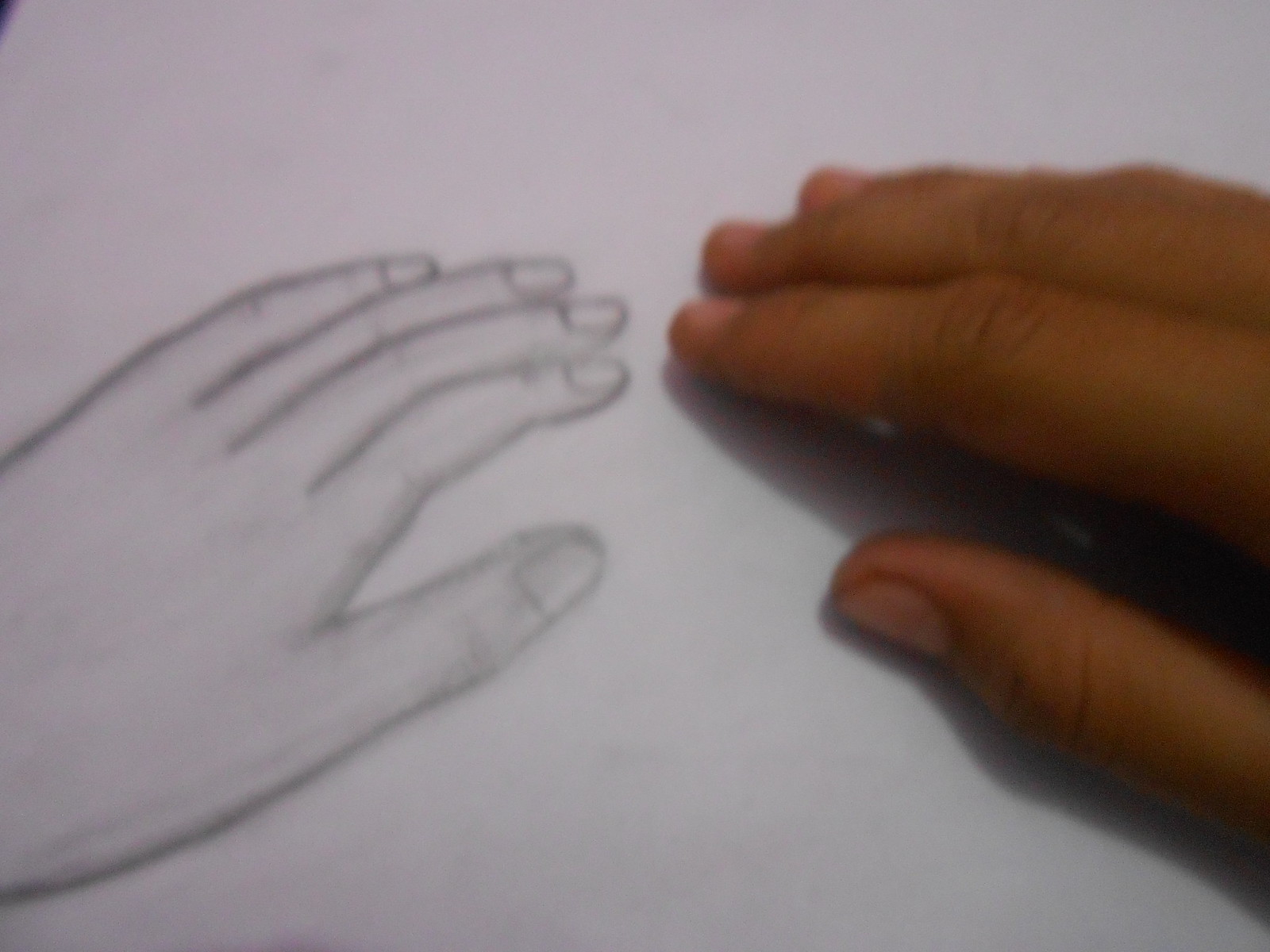The image, set against a gray background, showcases a juxtaposition of a real and a sketched hand. On the right side of the image, a person’s hand is visible, with only the thumb and three fingers on display, arranged as if resting on a surface. The skin of this hand appears dark or tanned, and the nails are short and neatly trimmed. This hand is partially depicted, with the wrist and top portion of the hand out of frame.  

To the left side, a hand drawn in pencil or gray chalk emerges from the bottom of the frame. This sketched hand is a detailed outline, displaying all four fingers and a thumb, positioned with the thumb at the bottom and the little finger towards the top. The drawn hand includes distinct knuckle details but remains unshaded, providing a stark, monochromatic contrast to the real hand beside it.